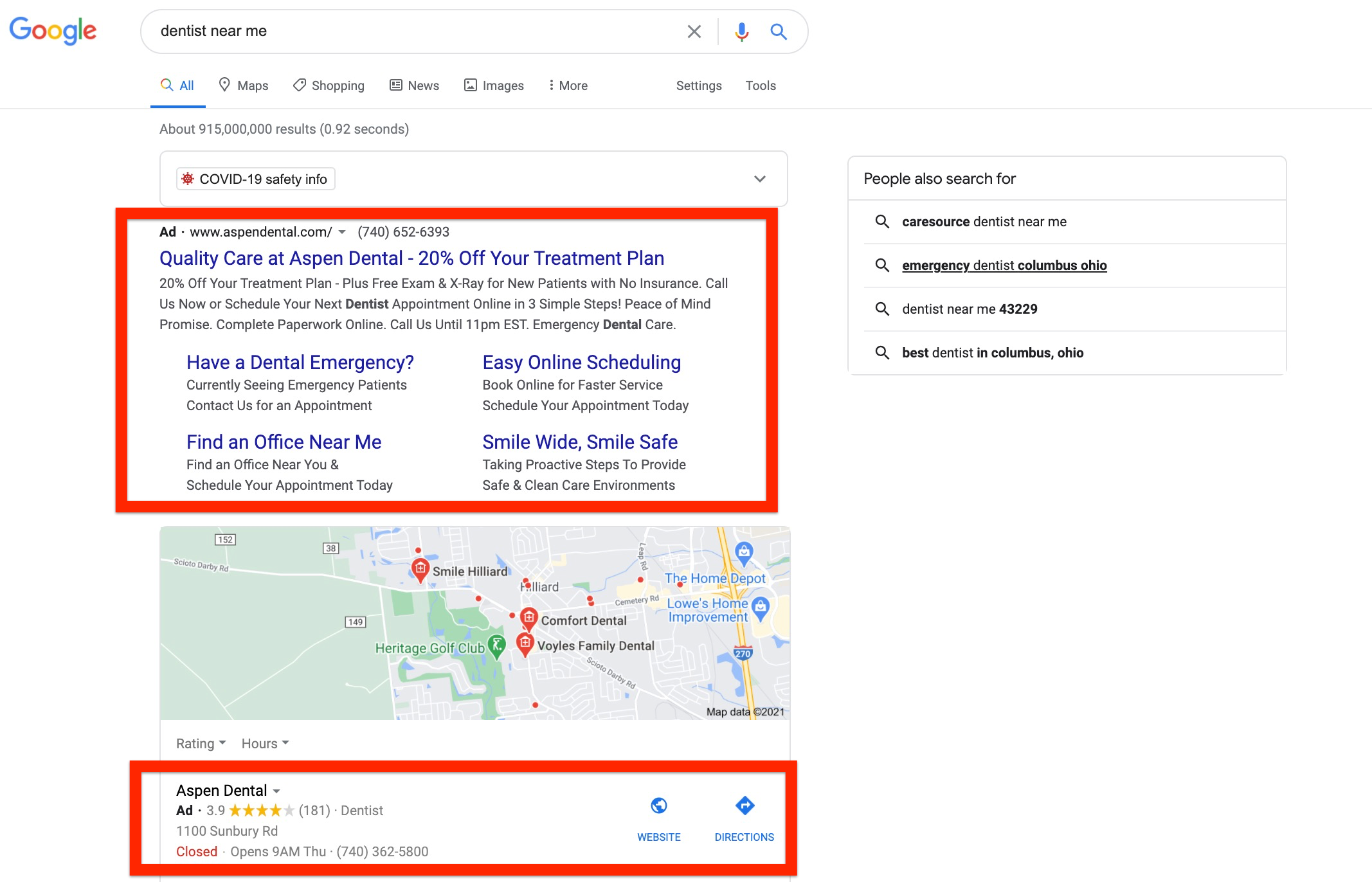This image captures a screenshot of a Google search result for "dentist near me," with the search query located at the top right of the screen beside the iconic, multicolored Google logo. Below the search bar, there are tabs for "All," "Maps," "Shopping," "News," "Images," and "More," accompanied by options for "Settings" and "Tools" on the far right. The search results indicate the total number of results and the time it took to generate them. 

Directly underneath this, a prominently placed banner provides "COVID-19 safety info," featuring a graphic of the COVID-19 virus with its characteristic spike proteins. The first search result is an advertisement for AspenDental.com, highlighted by a distinctive red rectangle to draw attention. 

Further down the page, a map displays several dental offices such as Smile Hilliard, Comfort Dental, and Voyles Family Dental, each marked with pins for easy identification. The map also highlights nearby landmarks, including Home Depot and Lowe's Home Improvement. Additionally, the map notes that these locations are on Sunbury Road. 

At the bottom, another section related to Aspen Dental offers clickable links for their website and directions, also emphasized by a red rectangle.